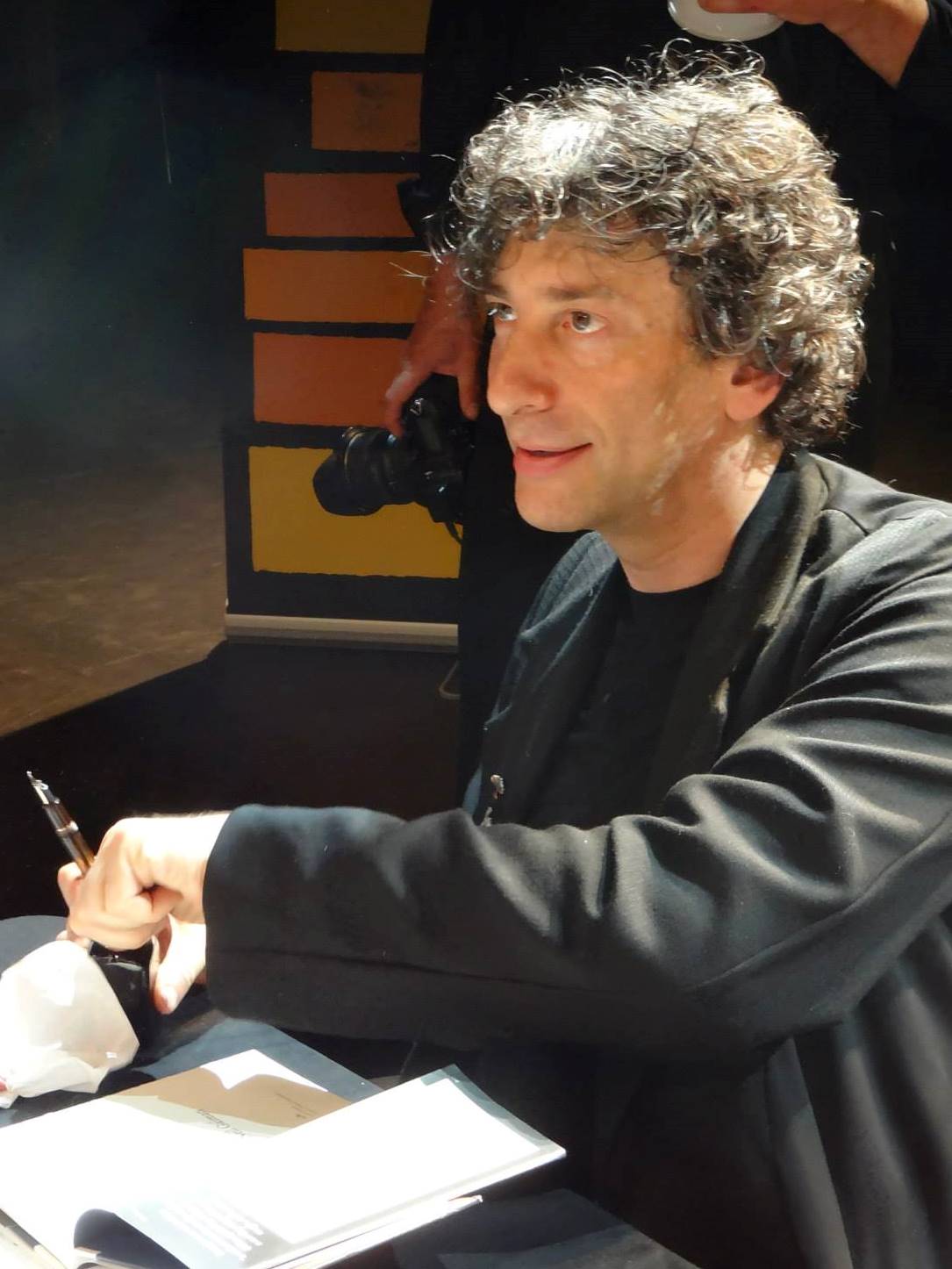In this image, a man resembling author Neil Gaiman is seated at a black desk. He has dark, wavy, and curly hair that extends past his neck, almost to his shoulders. Gaiman's complexion is tanned, and he wears a black long-sleeved jacket over a black t-shirt. His gaze is directed to the side, not directly at the camera. Before him lies an open notebook with two visible white pages, and he holds a brownish-black pen in his right hand, poised as if to sign the pages. In the background, a photographer dressed in dark clothing is seen, though only their right hand, gripping a black camera, is fully visible. Their left hand, also partially visible, supports the camera. On the wall behind the photographer, stacked colored shapes in yellow and orange hues add visual interest. This setting likely indicates an indoor book-signing event.